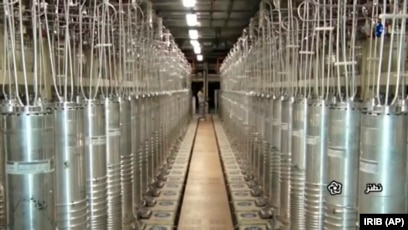The image is a detailed color photograph of an industrial warehouse or factory setting. Central to the composition is a long, dimly lit corridor that recedes into the distance, illuminated by industrial-style fluorescent lights overhead. On either side of this aisle are rows of tall, shiny metallic canisters, each approximately 4 feet in length and 1.5 to 2 feet in diameter. These canisters are tightly packed together and mounted on slightly elevated platforms. At the top of each canister, tubing or wiring extends upwards towards the ceiling. Although some canisters have symbols or stickers, these markings are not legible. Near the far end of the corridor, there appears to be a person standing close to a darkened doorway, possibly interacting with a panel stationed there. The dominant colors in the image include the silver sheen of the canisters, complemented by the contrasting beige, black, and the white tubing. In the bottom right corner, there is a black label with white uppercase lettering reading "IRIB (AP)."